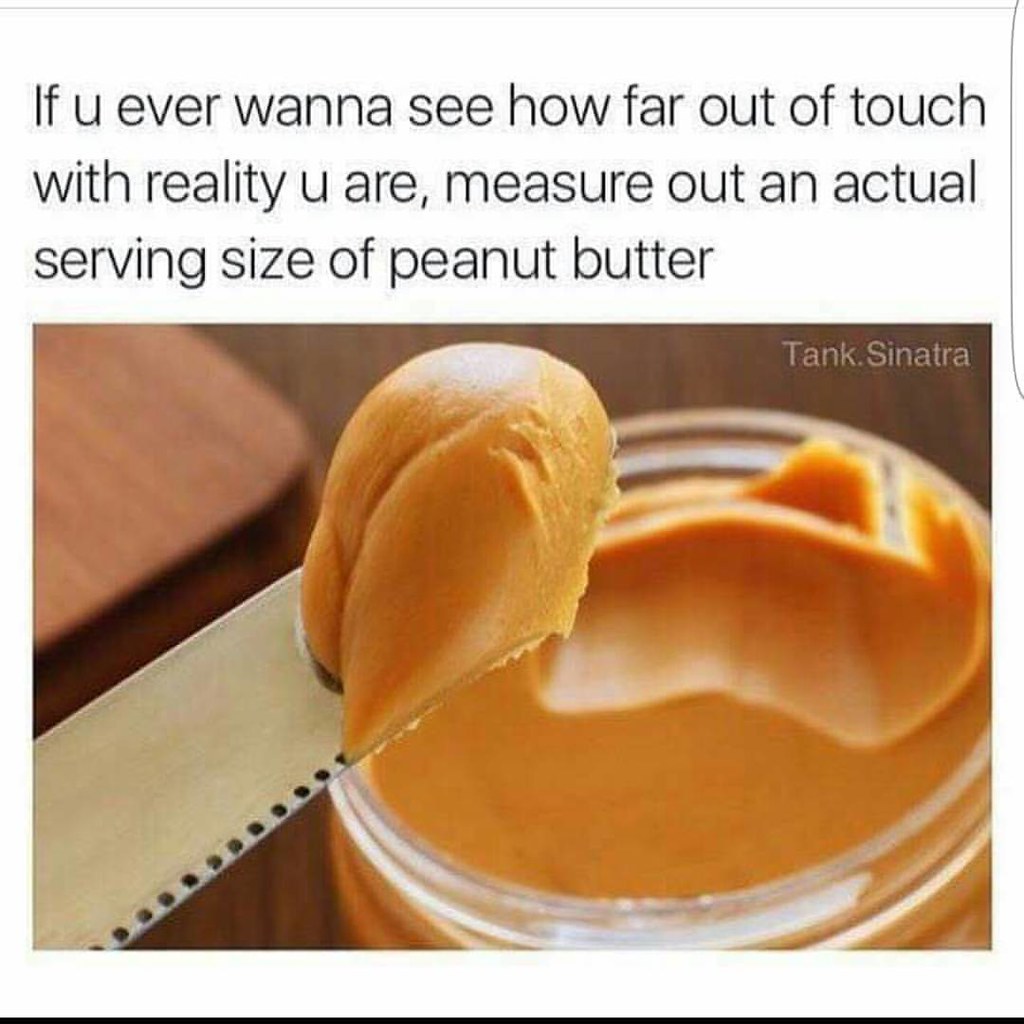This image appears to be a meme featuring a humorous take on serving sizes with a white top section containing black text that reads, "If you ever want to see how far out of touch with reality you are, measure out an actual serving size of peanut butter." The text is anchored by very thin black lines both at the very top and the very bottom of this section, with an interrupted black line running down the left side. Below the text, a color photograph shows an open jar of thick, brown peanut butter sitting on a slightly out-of-focus wooden table. A butter knife, positioned centrally, has scooped out a tiny portion of the peanut butter, barely covering its tip—this minuscule amount humorously highlights the absurdity of recommended serving sizes. In the upper right corner of the photo, "tank.Sinatra" is inscribed in gray text.